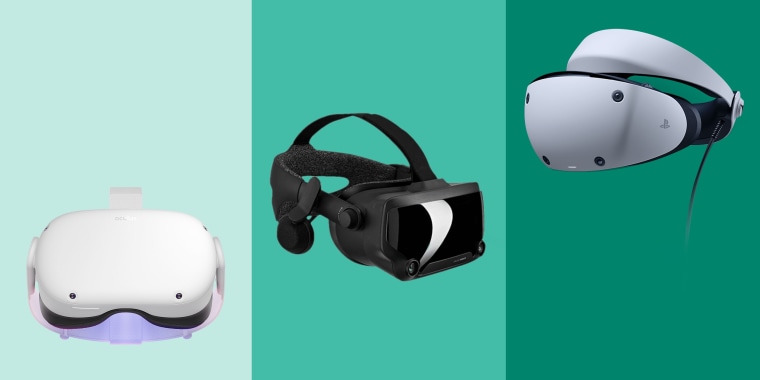These are three distinct images showcasing virtual reality goggles, each set against varying shades of green backgrounds. The first image, on the far left, features a white VR headset with black eyepieces placed against a pale turquoise background. The headset appears closed, offering minimal insight into its fitting mechanism. The middle photograph presents a black VR headset with ear pieces, a glossy black front shield, and a head cover, set against a medium turquoise to darker blue-green backdrop. This headset distinctly shows its straps designed to fit around the head, with one strap going over the top and another around the back. The final image on the right displays a white PlayStation VR headset with a futuristic design, notable black detailing on the front, and a visible cable extending from it. The background here is a rich forest green. Each quadrant emphasizes different aspects of the headsets against distinct green hues, providing a comparative view of design and structure.